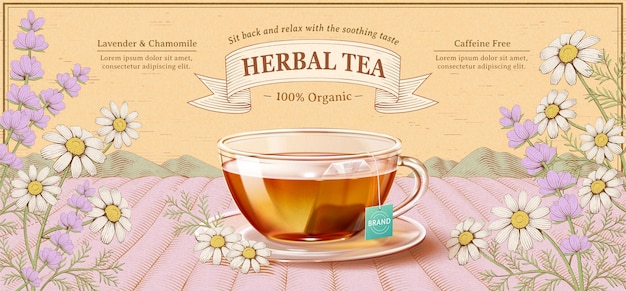This image appears to be an illustrated mock-up of a herbal tea box, featuring a serene and picturesque setting. The dominant visual element is a clear glass cup filled with a honey-colored tea and a visible teabag, labeled with a generic "brand" tag, suggesting a customizable branding option. The cup rests on a glass saucer, placed upon an artistically rendered lavender field with rolling hills and a pastel sky, which transitions from a peach color to blue, giving a tranquil atmosphere.

Above the cup, in the center, a beige banner with the words "Herbal Tea" written within a darker brown background stands out. Flanking this banner on both sides are the phrases "100% Organic" with decorative dashes. The tagline "Sit back and relax with a soothing taste" appears above the banner in a lighter shade that could be dark gray or dark brown. Additional texts, "Lavender and Chamomile" placed at the top left and "Caffeine Free" on the right, are written in gray, indicating the tea's ingredients and its caffeine-free nature. All these elements are set against a soft, beige-colored background, adorned with daisies with yellow centers and purple lavender flowers, adding to the overall calming aesthetic. The combination of these detailed visual and textual elements suggests this is a meticulously designed template for an herbal tea product, aimed at evoking a sense of relaxation and natural purity.